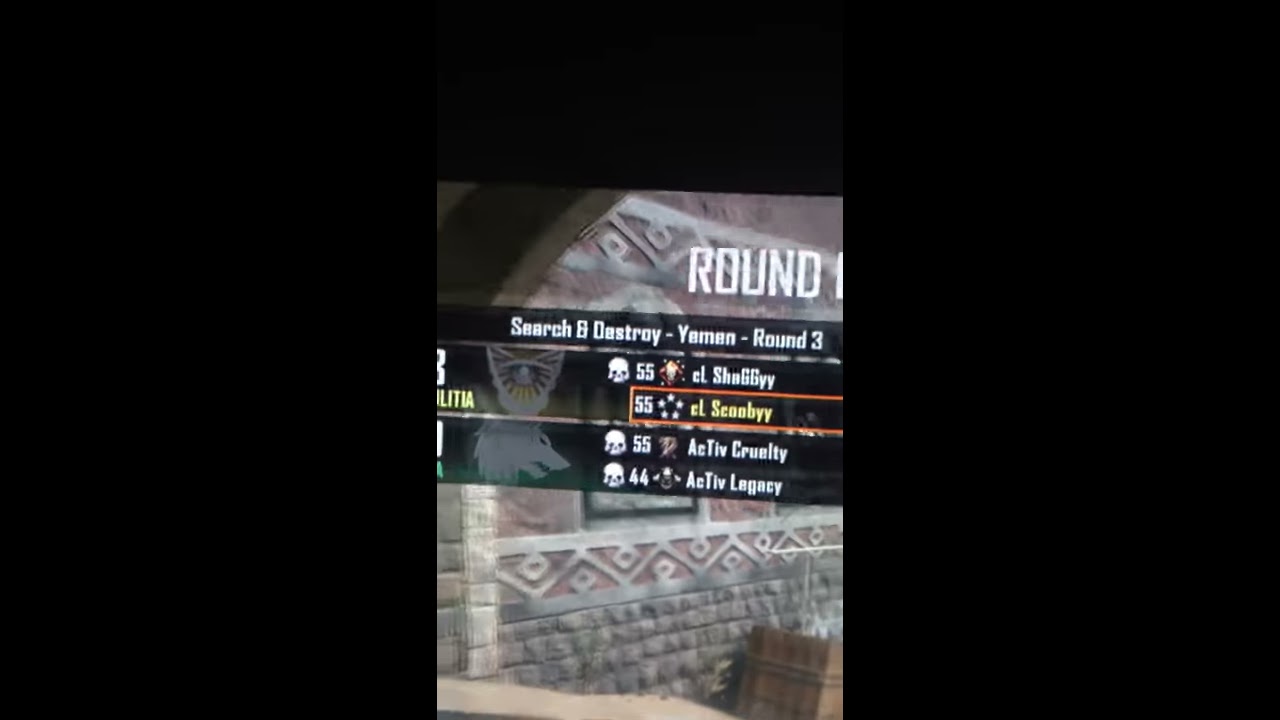This is a detailed screenshot from a video game reminiscent of Call of Duty. The primary image features a stone wall with distinctive geometric designs, including gray bricks at the bottom and a reddish plaster overlay with zigzag and diamond patterns above. A gray arched window is also visible. The screen is bordered on the left, right, and top, with the borders occupying significant portions of the image. In the center, overlapping the wall, are game details in white text on black banners: "Round 1," "Search and Destroy Yemen Round 3." There are four player names listed vertically, each accompanied by a number and skull icons, indicating their statuses: El Shaggy (skull, 55), El Scooby (55), Active Cruelty (skull, 55), and Active Legacy (skull, 44). The numbers likely represent points or kills, suggesting El Scooby as the victor with no skull next to their name.